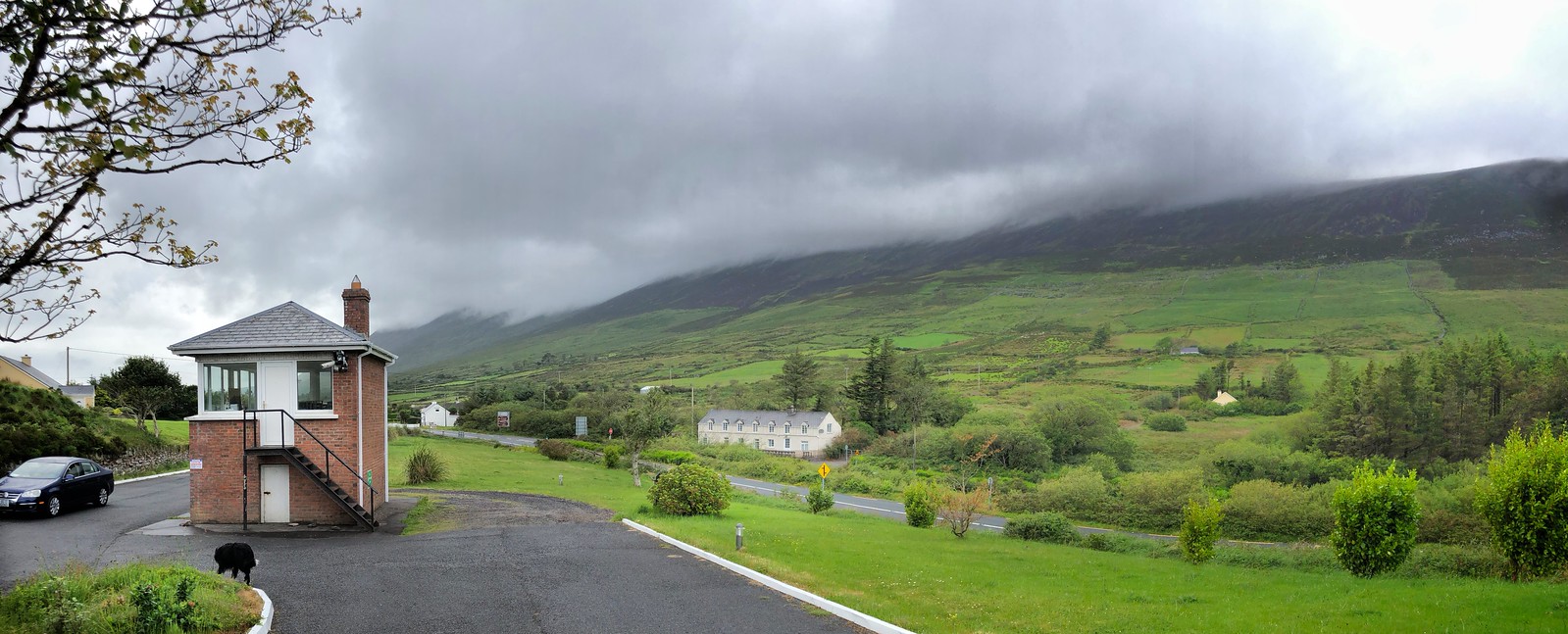The image depicts a picturesque landscape primarily characterized by a bright green hillside that slopes gently from right to left. Dominating the right side of the scene, this lush green slope is topped with a darker, mountainous hill. Above these hills, a vast gray storm cloud looms, contrasting against a predominantly whitish sky mixed with hints of blue and gray hues.

Nestled on the slope is a long, white two-story house with a gray roof, surrounded by trees and bushes. This idyllic rural setting continues with a road that curves around the hillside, leading to the left side of the image. Here, at the left edge, stands a small outpost or checkpoint building made of red brick with a gray roof and a black staircase ascending to its second floor. Adjacent to this building is a driveway where a black sedan is parked. In the vicinity, a black dog can be seen near the road.

The entire landscape evokes a tranquil yet dramatic atmosphere, possibly reminiscent of the English or Scottish countryside, with its vibrant grassy fields and overcast sky. The presence of these buildings, the curving road, and the detailed natural scenery contribute to a serene but dynamic rural tableau.